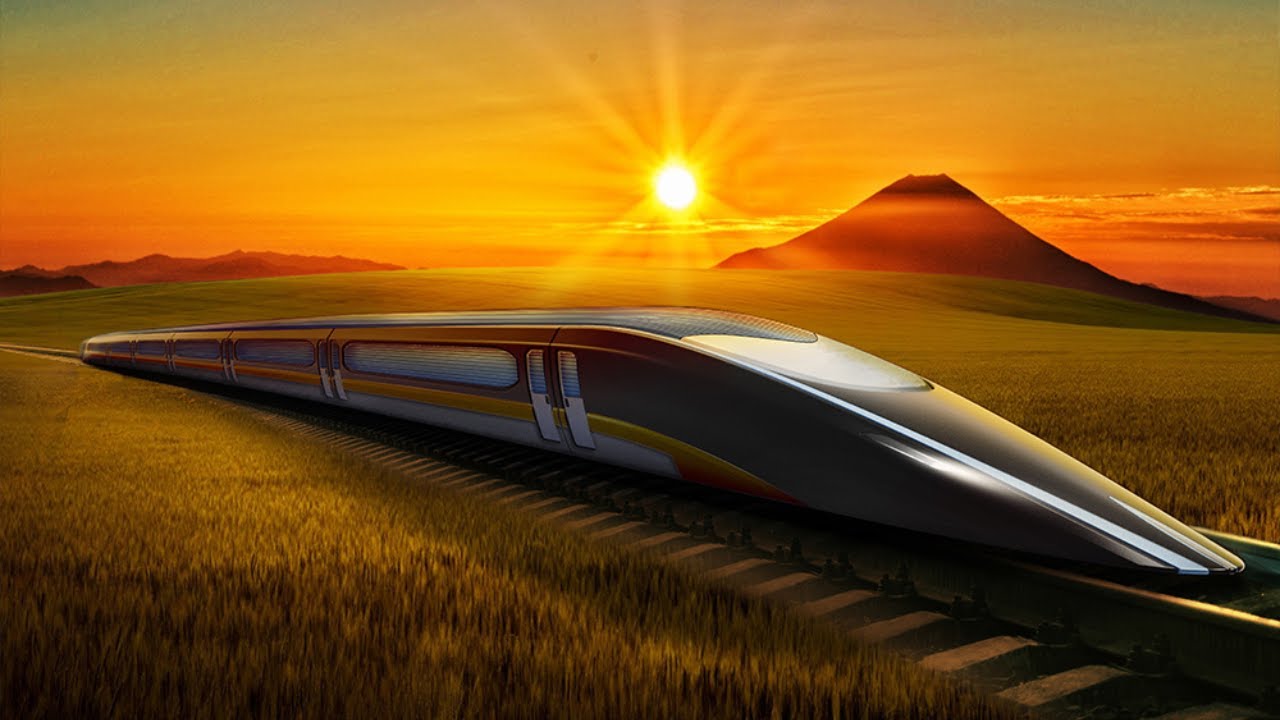The image depicts a digitally rendered painting, possibly created using AI, showcasing a sleek, aerodynamic bullet train racing along a railway track. The train, primarily gray with gold accents and white doors, features a long, slender front resembling a bird’s beak. The railway is surrounded by lush, green grass in the foreground. Beyond the grassy field, there are brown mountains, adding depth to the landscape. The background sky is predominantly yellow and orange, illuminated by a bright, round, white sun with radiant yellow rays. The sun appears to be setting, casting a warm glow over the entire scene and enhancing the golden hue of the sky.